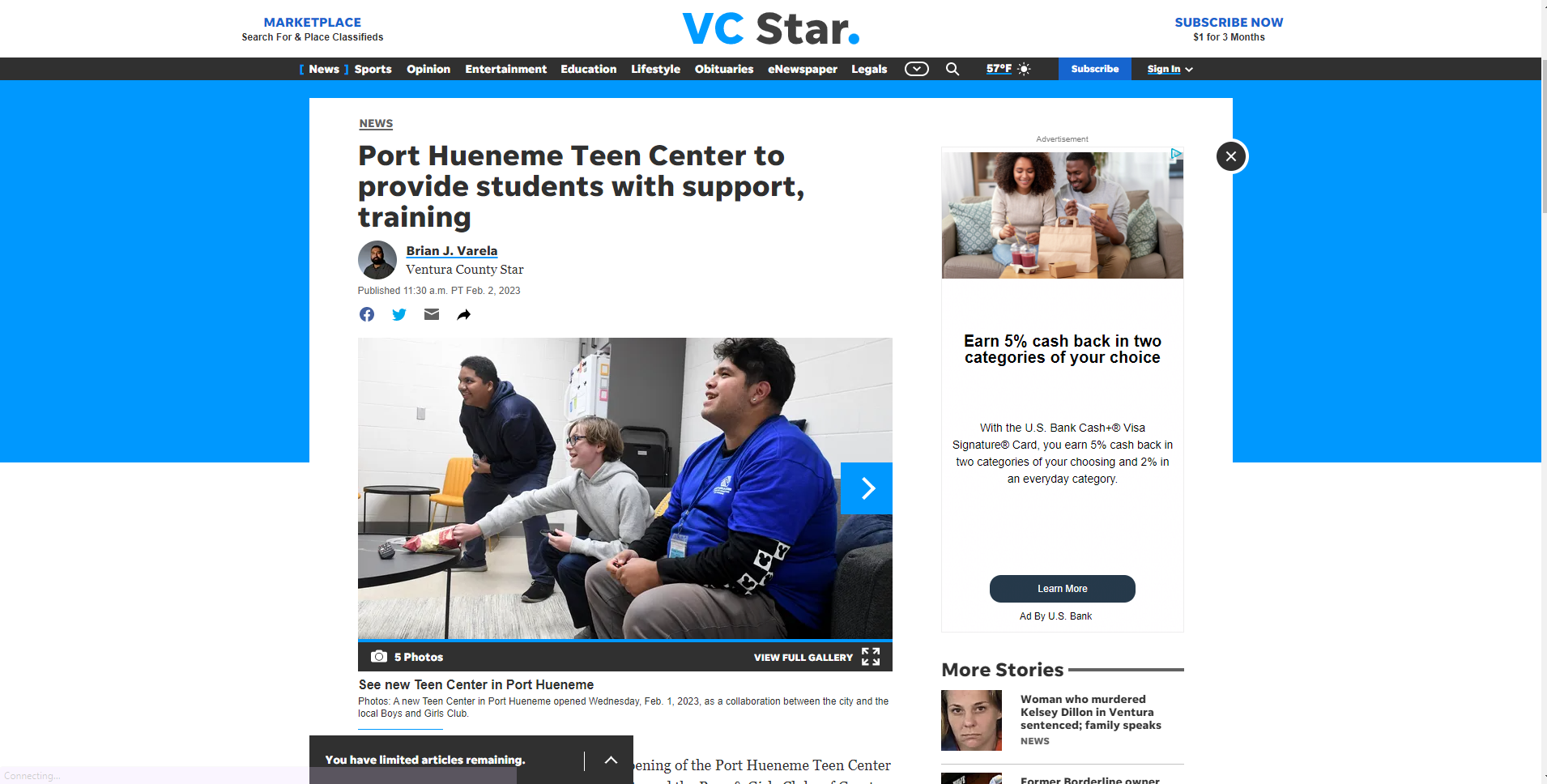This is a photo of a website, featuring a clean and organized layout. At the top, there is a white border, and about an inch from the left, another white border continues down the length of the page. The top-left corner prominently displays "MARKETPLACE" in bold, blue, all capital letters. Below that, in smaller black text, it reads "Search for In-place Classifieds."

Centrally, the website features "VC" in large blue capital letters followed by a black star symbol and a blue period. To the right of this, in blue, all capital letters, reads "SUBSCRIBE NOW," and directly underneath, the text notes "$1 for 3 Months" in black.

A black border separates sections of the site. The navigational menu, comprised of clickable sections, includes options in white and various colors: News, Sports, Opinion, Entertainment, Education, Lifestyle, Obituaries, E-Newspaper, and Legals. There is also a downward-pointing arrow tab, a search icon, and the current temperature displayed at 57 degrees Fahrenheit. To the right of the search bar, a blue tab reads "Subscribe" in white, and "Sign In" in an underlined blue font.

The midsection background transitions to a light blue, while the bottom half of the page is white. At the heart of the page, a newspaper tab pops up. In the top-left corner of this tab, “NEWS” is written in black, underlined text, followed by the headline "Port Hueneme Teen Center to Provide Students with Support and Training."

In the accompanying image, a profile picture of the author, Brian J. Varela, is shown. He has black hair, a green shirt, and a blue background. To the right of his picture, "Ventura County Star" is displayed, under which the publication date appears. Adjacent to these elements are the Facebook, Twitter, email, and share icons.

Beneath the headline, three individuals are seen playing video games in a room with a black table in front of them. Two sit on a brown couch, while one stands. In the top right corner, an African-American couple sits on a brown couch with blue pillows.